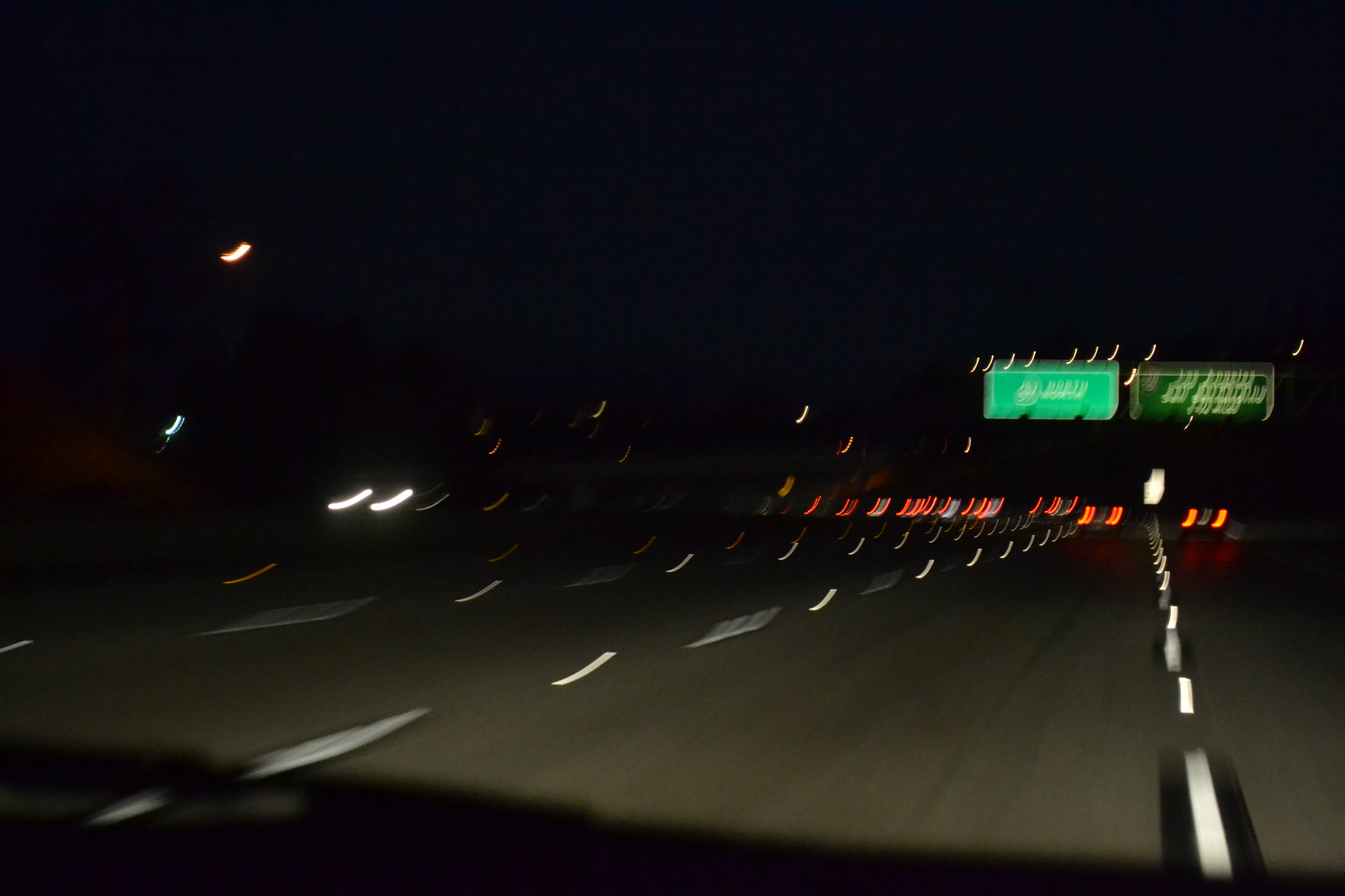The image is a highly blurry nighttime photograph of what appears to be a multi-lane highway, possibly an interstate, featuring four distinct lanes marked by dashed white lines. In the distance, there are several red lights, presumably the taillights of vehicles, spaced rhythmically apart, indicating a flow of traffic. The green highway signs are prominently visible but too out-of-focus to discern any text. One of these signs potentially bears the recognizable crest of the U.S. interstate system. The overall scene is immersed in darkness, with no visible stars, suggesting an overcast night sky.